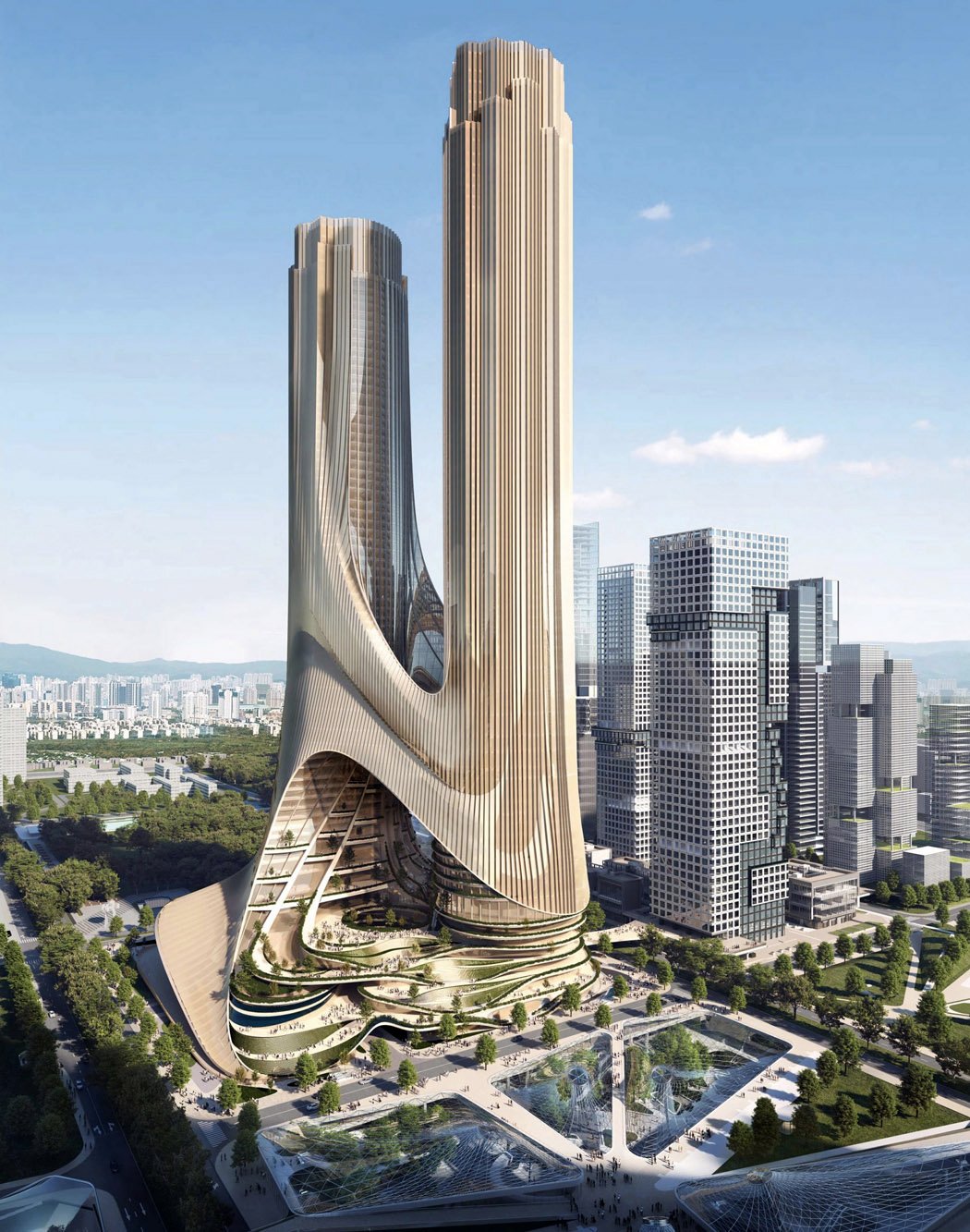The image is a striking, detailed artist's rendition of a futuristic cityscape, set on a sunny day under a clear blue sky that deepens to a richer blue at the top. Dominating the center is a massive, modern building with an imaginative design, resembling a U or Mu symbol. This building comprises two interconnected sections: a taller right tower with vertical beige and white lines, tiered at the top, and a shorter left tower, both adorned with numerous small windows. The structure is further enhanced by layered, balcony-like terraces, that include gardens and greenery at various levels, lending a surreal and dreamlike quality.

Below the imposing towers are roadways and walkways lined with neatly planted trees, contributing to the well-maintained, clean appearance of the urban environment. Tiny people can be seen as dots, emphasizing the impressive height of the observation point. Surrounding this architectural marvel are several other rectangular, silver skyscrapers filled with windows, creating a bustling cityscape. The scene evokes a sense of advanced urban planning, blending modern architectural styles with natural elements, set against a backdrop of smaller buildings and a serene sky.